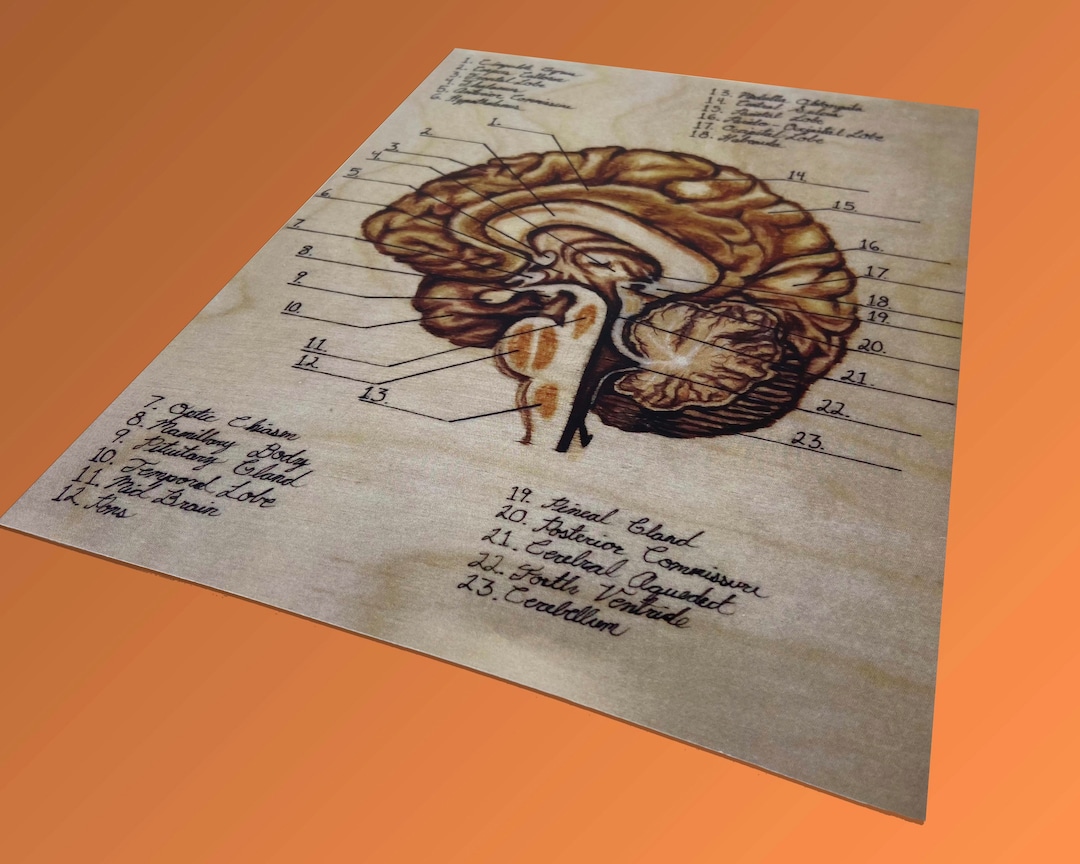The image is a detailed, brown and white illustration of a sagittal section of the brain, similar to what you would find in a textbook or a finely crafted wood carving with wood-burning details. The brain is cut in half, revealing its internal structures, and is meticulously labeled with numbers ranging from 1 to 23. Black lines extend from each number to specific parts of the brain, and the corresponding labels are written in black cursive text. Among the numbered labels, notable parts include the optic chiasm (7), mammillary body (8), pituitary gland (9), temporal lobe (10), midbrain (11), pineal gland (19), posterior commissure (20), cerebral aqueduct (21), fourth ventricle (22), and cerebellum (23). The numbers 1 through 13 are listed on the left side of the brain, while 14 through 23 are on the right. The brain illustration appears at a slight angle, providing a somewhat three-dimensional perspective, with an orange background accentuating its anatomical details.